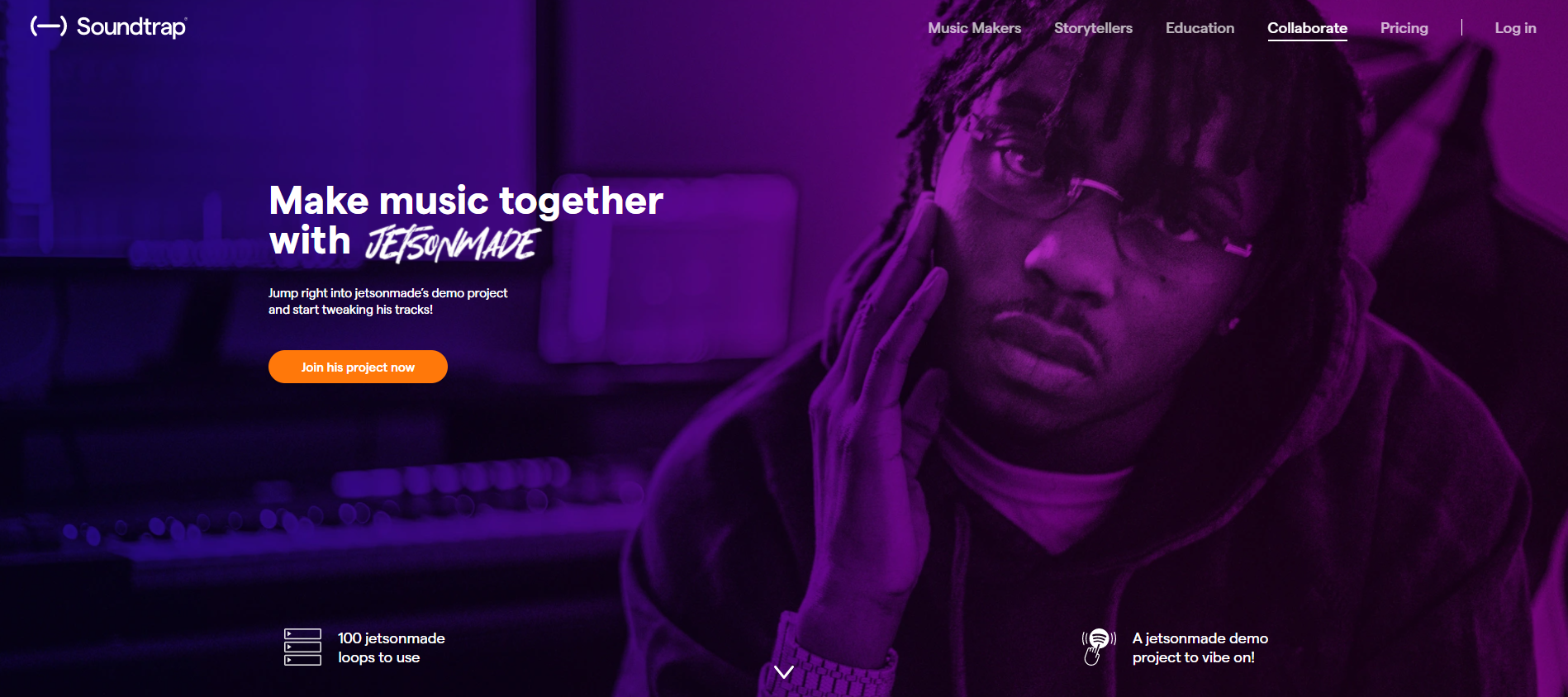Screenshot of a web page featuring an image and interface elements. At the top of the screen, it displays the text "Soundtrap" with a minus sign in parentheses beside it. The prominent image shows an African-American man with glasses and braided hair, his hand raised thoughtfully to the side of his face. He is wearing a hoodie over a white t-shirt and has a stylish watch on his wrist. The background transitions from a bluish-purple hue on the left to solid purple on the right, with what appears to be a musical keyboard partially visible. Overlaying this image in white text is the phrase, "Make music together with JetsonMade." Toward the bottom of the screen, there is an orange "Join" button located near a keyboard area. Additional text in this section includes "100 JetsonMade" and some blank clickable areas. The top of the page features dropdown menus for navigation options.